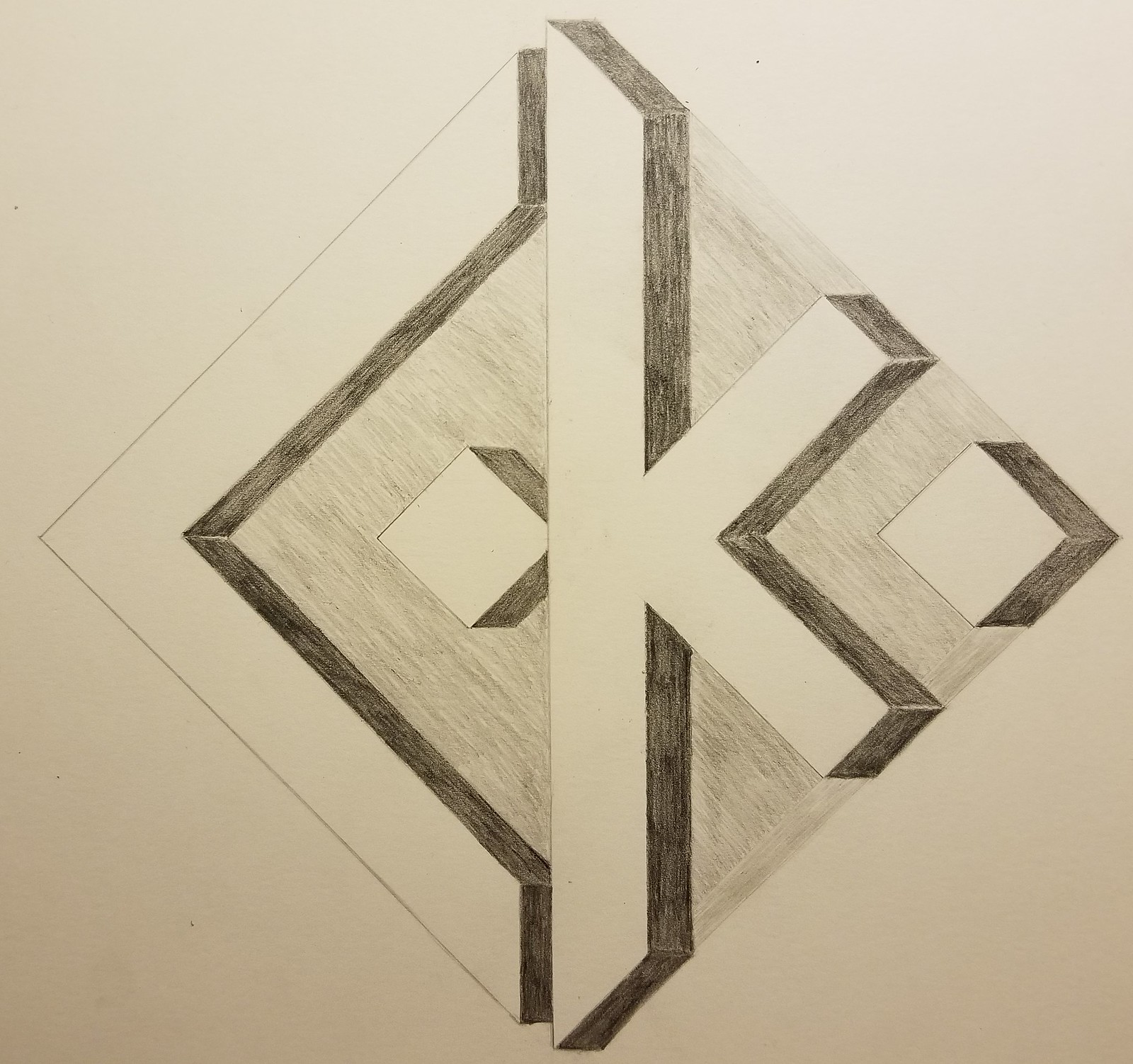This image is a detailed pencil sketch on white paper, illustrating a complex and abstract geometric composition. On the left side of the sketch, there is a shape resembling a less-than sign ("<"). Adjacent to this shape on the right, there is a structure that looks like a modified letter "K," where the diagonal strokes are shortened. Attached to the right side of this "K" shape is a three-dimensional cube, and another cube is connected to the middle vertical segment of the "K."

Each object in the drawing is depicted in three dimensions, with careful shading to emphasize their prismatic forms. The entire composition sits on a square base, lightly shaded in a soft gray, adding depth and grounding the abstract geometric arrangement in its space.